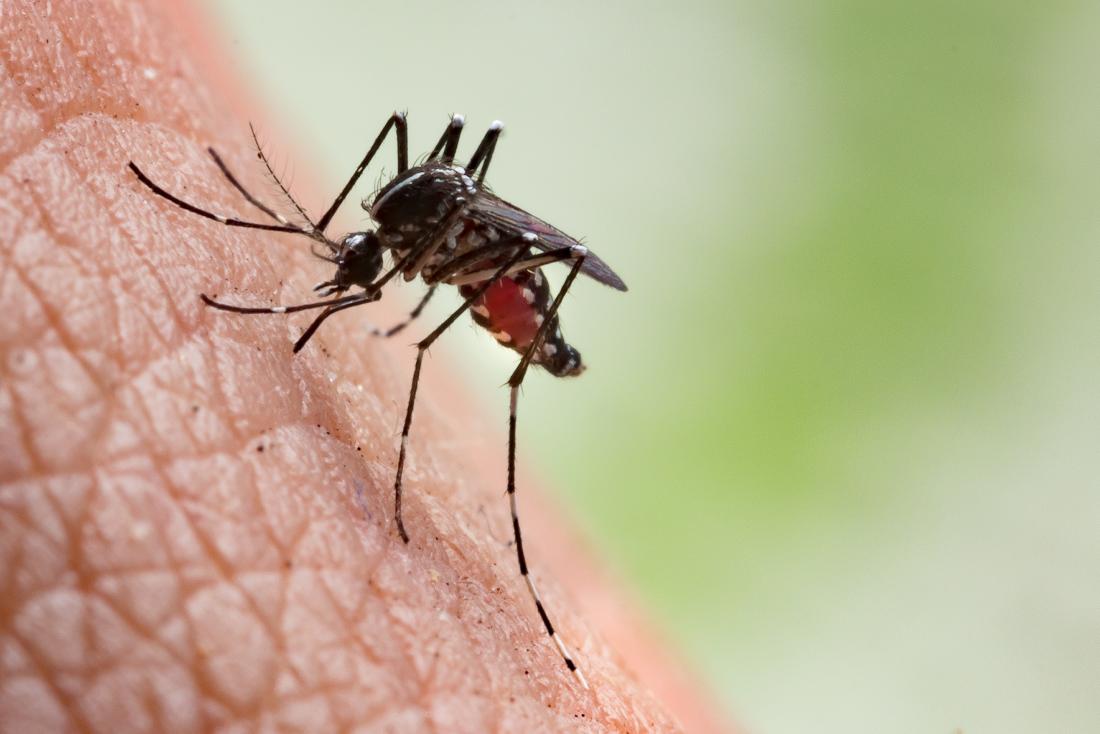The image is a highly magnified digital photograph showcasing a close-up view of a mosquito actively biting human flesh. The left diagonal side of the picture captures the Caucasian person's skin, which is segmented with visible lines, indicating a significant zoom level. The mosquito, centrally positioned, is predominantly black with distinct white stripes on its head and back, as well as white spots on its head, belly, and legs. Notable is its red underbelly, engorged with blood. The insect's long, spindly legs extend from its body, and two prominent projections, likely its mouthparts, penetrate the skin. Behind the mosquito, the blurred background displays a white color with a greenish stripe descending from the upper right corner to the center, enhancing the focus on this intense moment.